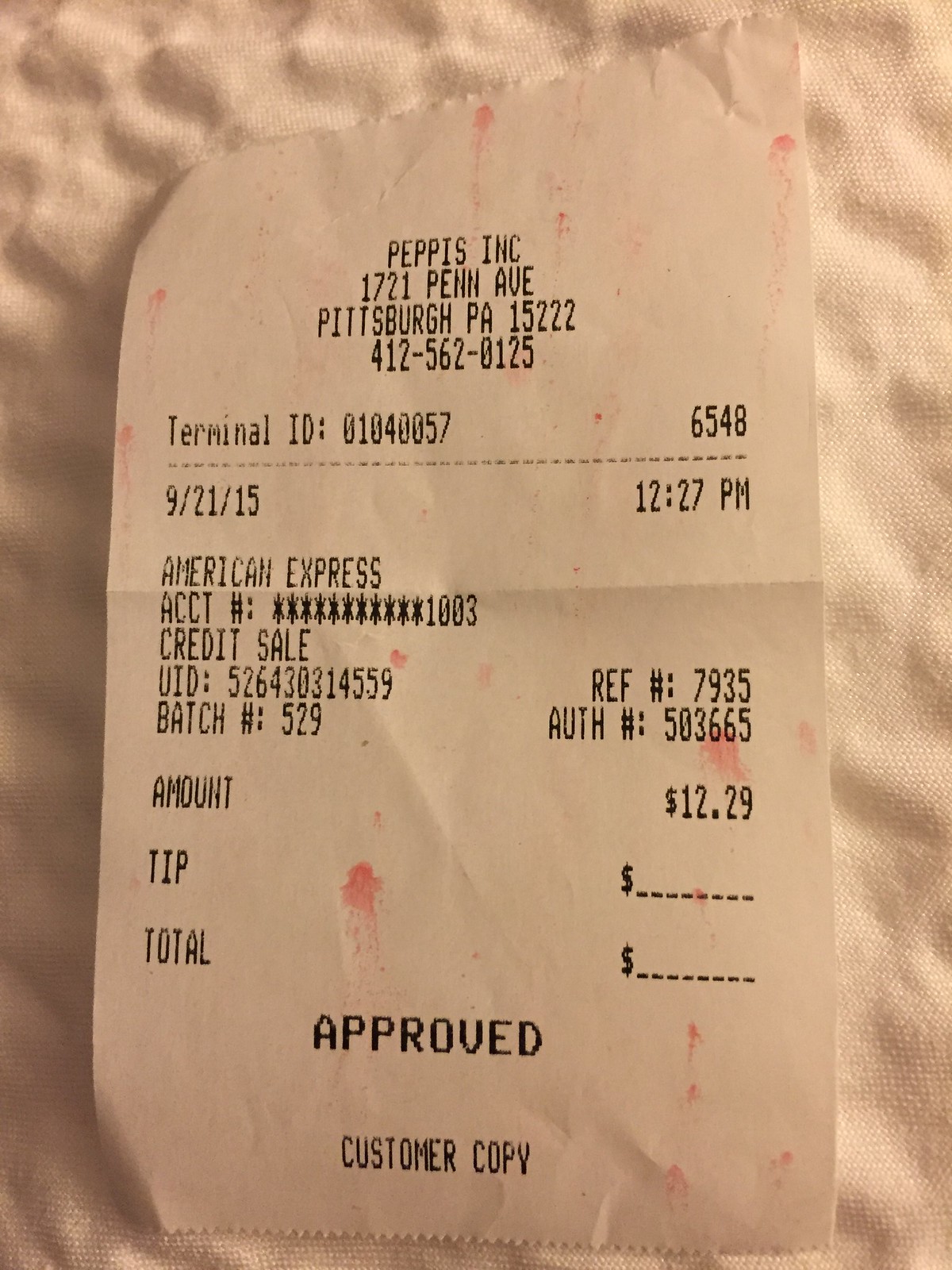The image features a beige fabric backdrop with a slightly off-white receipt placed on top. The receipt is fully visible, with all text printed in black. The header reads "Peppis, Inc." followed by the address "1721 Penn Avenue, Pittsburgh, PA 15222" and the phone number "412-562-0125." Below this, the receipt lists a "Terminal ID" as "0104-0057." The transaction details show an American Express card with the account number ending in "1003" was used for a sale amounting to "$12.29." The date and time of the transaction are specified as "9-21-2015" at "12:27 PM."